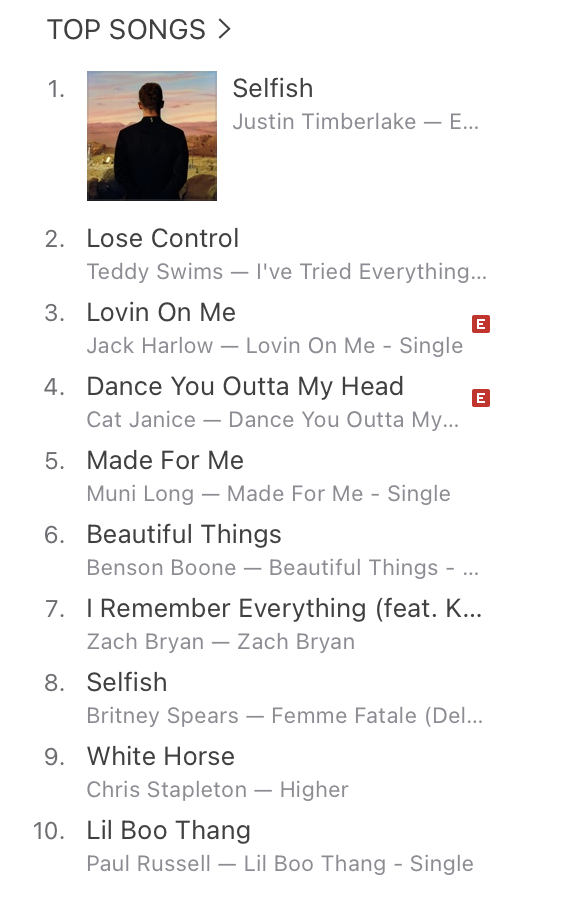The image displays a list of the top 10 songs under the heading "Top Songs" positioned in the top left corner. The detailed list is as follows:

1. "Selfish" by Justin Timberlake
2. "Lose Control" by Teddy Swims
3. "Loving on Me" by Jack Harlow (Loving on Me Single)
4. "Dance You Out of My Head" by Kat Janis (Dance You Out of My Head)
5. "Made for Me" by Mooney Long (Made for Me Single)
6. "Beautiful Things" by Benson Boone (Beautiful Things)
7. "I Remember Everything" by Zach Byer & Zach Bryan
8. "Selfish" by Britney Spears (Femme Fatale)
9. "White Horse" by Chris Stapleton (Higher)
10. "Lil Boothang" by Paul Russell (Lil Boothang Single)